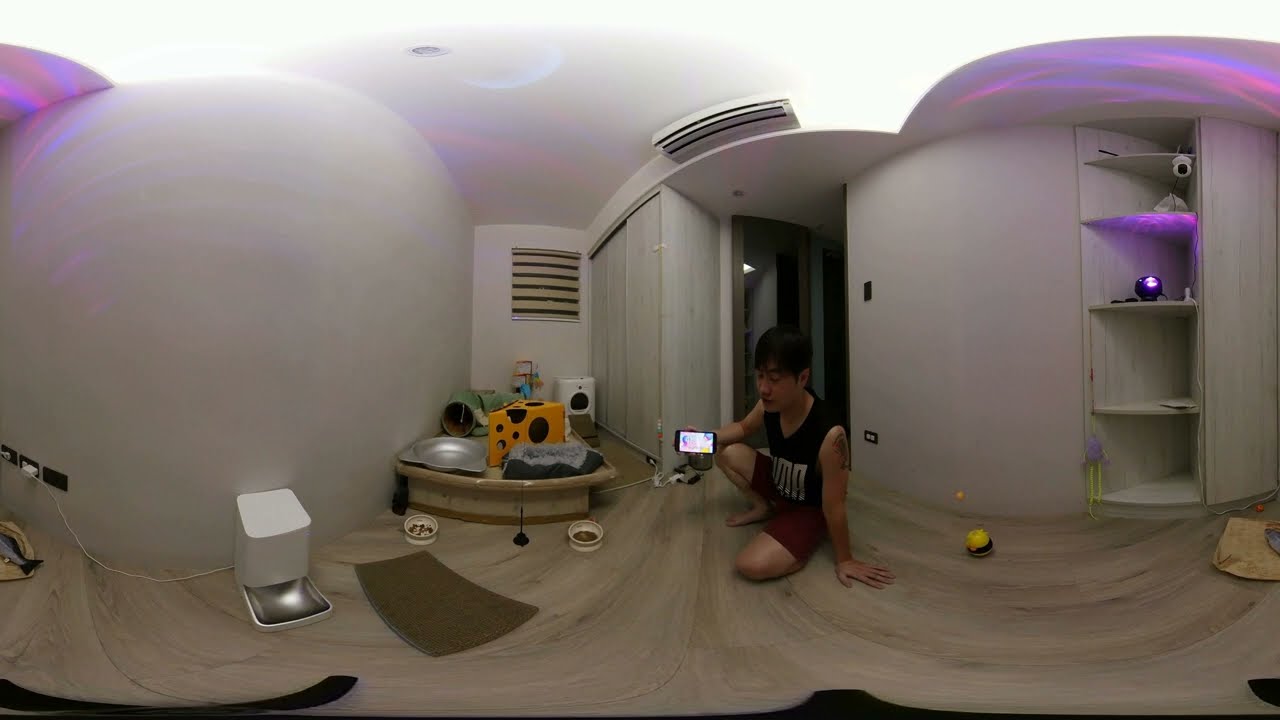The photo depicts the interior of a room evidently set up for cats, showcasing a combination of feline amenities and modern comforts. Dominating the left side is a white automated pet feeder, adjacent to which lies an array of cat toys, including a giant block of cheese with holes for crawling and a miniature tunnel. In front of the toys are two food bowls placed on a small mat. Kneeling on the lighter-colored hardwood floor, slightly to the right of center, is an Asian man with short black hair, dressed in a black muscle shirt emblazoned with the Puma logo, and dark red shorts. He is holding a smartphone in landscape orientation, presenting its screen to the viewer. The man’s left bicep displays a visible tattoo. Further to the right, built-in shelves line the white, subtly curved walls; one of these shelves supports a black spherical projector, while another holds a white webcam. A strobe light is also noticeable on a different shelf. At the very back of the room, a white litter box sits under a small window adorned with a tan shade. A closed closet door is also discernible in the background.